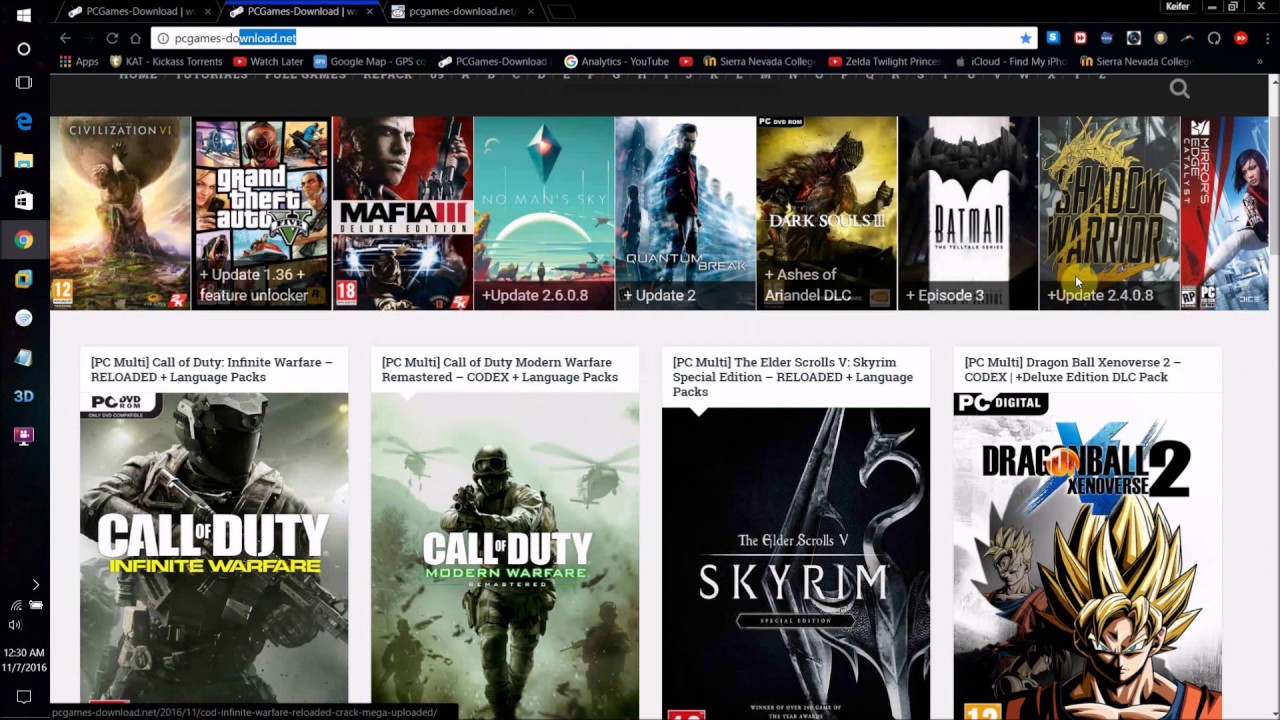A screenshot from a computer screen showcasing a webpage for downloading PC games. At the top, a black border frames the screen, below which a white address bar is visible with the search term "PC games download" typed in. To the far right of the address bar, a blue star icon is present. Below the search bar, there is a row of nine video game covers displayed prominently. The games featured include popular titles such as Civilization, Grand Theft Auto, Mafia 3, and others. One cover depicts a sky background with a moon and a diamond, the title of which is not clear. Other recognizable covers include Quantum, Dark Souls, Batman, and Shadow Warrior. The ninth cover is partially cut off, showing a fighter against a blue background. On the left side of the screen, there is a vertical column of icons for various applications, including Internet Explorer, a file icon, Google Chrome, an icon labeled "3D," and one resembling a clock. At the bottom of the screen, four additional game titles are visible: Call of Duty: Infinite Warfare, Call of Duty: Modern Warfare, Skyrim, and Dragon Ball Xenoverse 2.